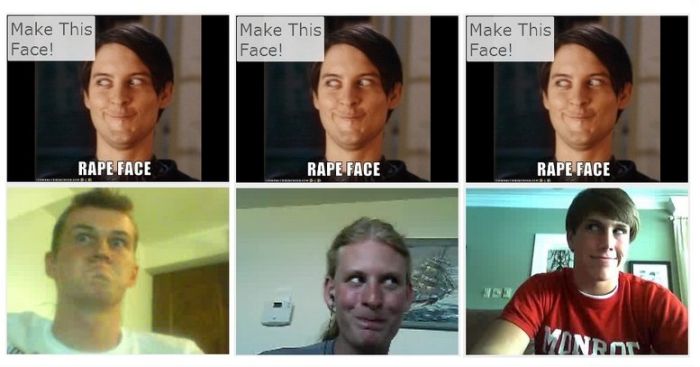The composite image consists of six individual pictures arranged in two rows. The top row features three identical images of the same man. Each of these images has a small gray rectangle in the upper left corner with black text that reads "MAKE THIS FACE!" In these images, the man is rolling his eyes all the way to his right and keeping his mouth closed, displaying an exaggerated expression. Additionally, there is text in white capital letters placed on the leg area of the man that reads "RAPE FACE."

The bottom row showcases three different people. The first individual, positioned on the bottom left, is a man with long hair wearing a white t-shirt, standing in front of a brown door. His facial expression conveys disgust, with his eyes looking off to the side and his mouth closed. The middle image is of a woman with a middle hair part, dressed in a gray t-shirt, and standing in front of a white wall adorned with a drawing of a ship and a thermostat. She mirrors the expression by also darting her eyes to the left and closing her mouth. Lastly, the bottom right image features another man wearing a red t-shirt with the white letters "MONROE" (spelled out as M-O-N-R-O-E). He is slightly grinning while rolling his eyes to the right. Two framed pictures are visible on the gray wall behind him, completing the scene.